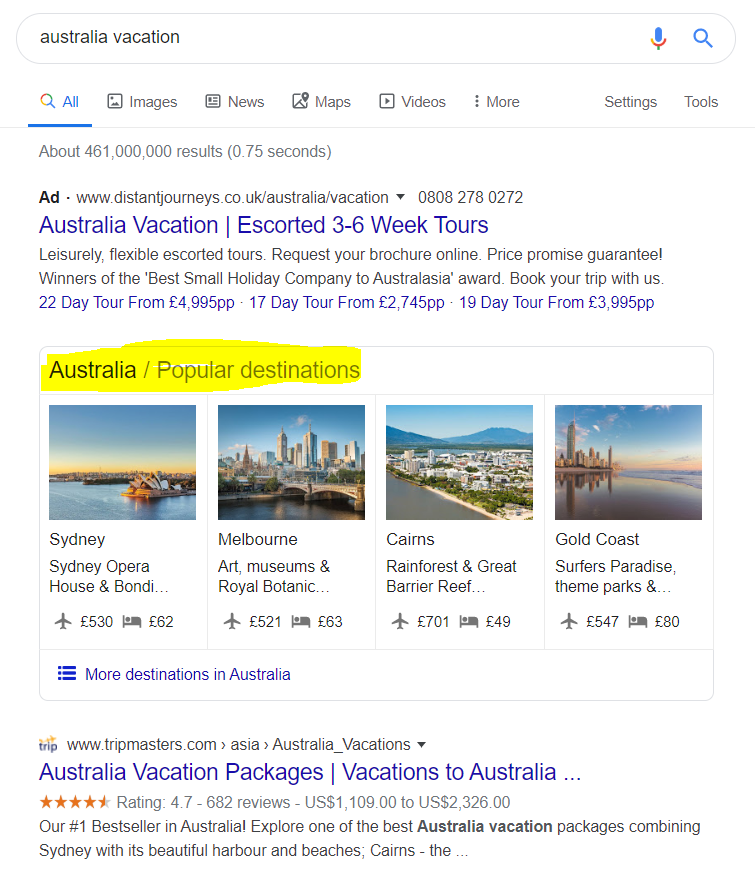Portrait-mode screenshot of a Google search results page featuring vacation options to Australia. The background is predominantly white, with the Google search bar situated at the top, followed by category headers, with "All" being selected.

The first listing is an advertisement for "Australia Vacation Escorted Three to Six Week Tours." Below this ad, there's a highlighted section marked in yellow by the person who took the screenshot. This section is titled "Australia / Popular Destinations" and features four destinations: Sydney, Melbourne, Cairns, and the Gold Coast, each accompanied by an image of the respective location.

Each destination entry shows a detailed description, an airplane icon listing prices in British pounds for flights, and a hotel icon listing accommodation prices in British pounds. At the bottom of this section, there's a blue "More destinations in Australia" link with three horizontal menu lines next to it.

Following this, there's a segment not marked as an ad featuring Tripmasters. It includes a Tripmasters icon along with "Australia Vacation Packages" text, providing an overview of vacation options in Australia, accompanied by ratings and descriptions.